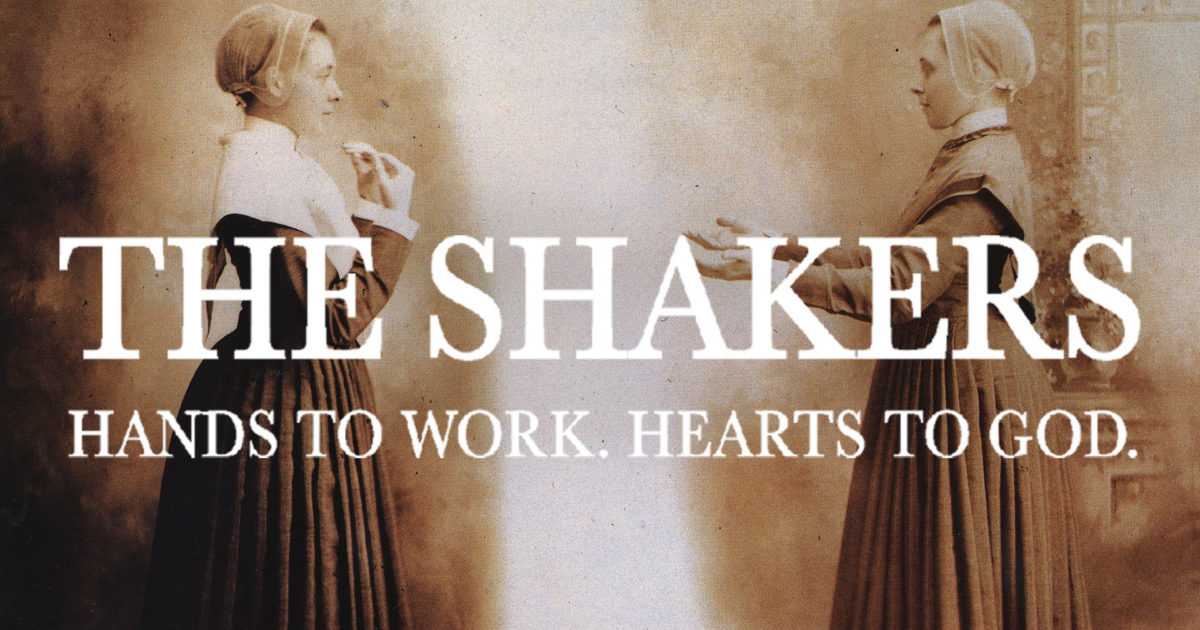This black-and-white sepia-toned photograph depicts two teenage Shaker women, probably around 15 or 16 years old, dressed in full-length dresses from the 1800s to early 1900s. The dresses appear to be black due to the monochromatic nature of the image, and both women are wearing shawls or capes over their dresses. They have bonnets on their heads, each adorned differently; one with a lined circular design and the other with a simpler, bordered style. The woman on the right extends her arms outwards, while the woman on the left bends her elbows with her fingers outstretched towards herself, creating an inviting gesture. Their plain faces and direct gazes towards one another enhance the historical atmosphere. The background is indistinct and features vague hints of a room with molding and wallpaper, fading into darker tones at the edges. Overlay text in large white capital letters reads "The Shakers," followed by "Hands to Work. Hearts to God." in slightly smaller uppercase letters, promoting the Shaker community and its values.